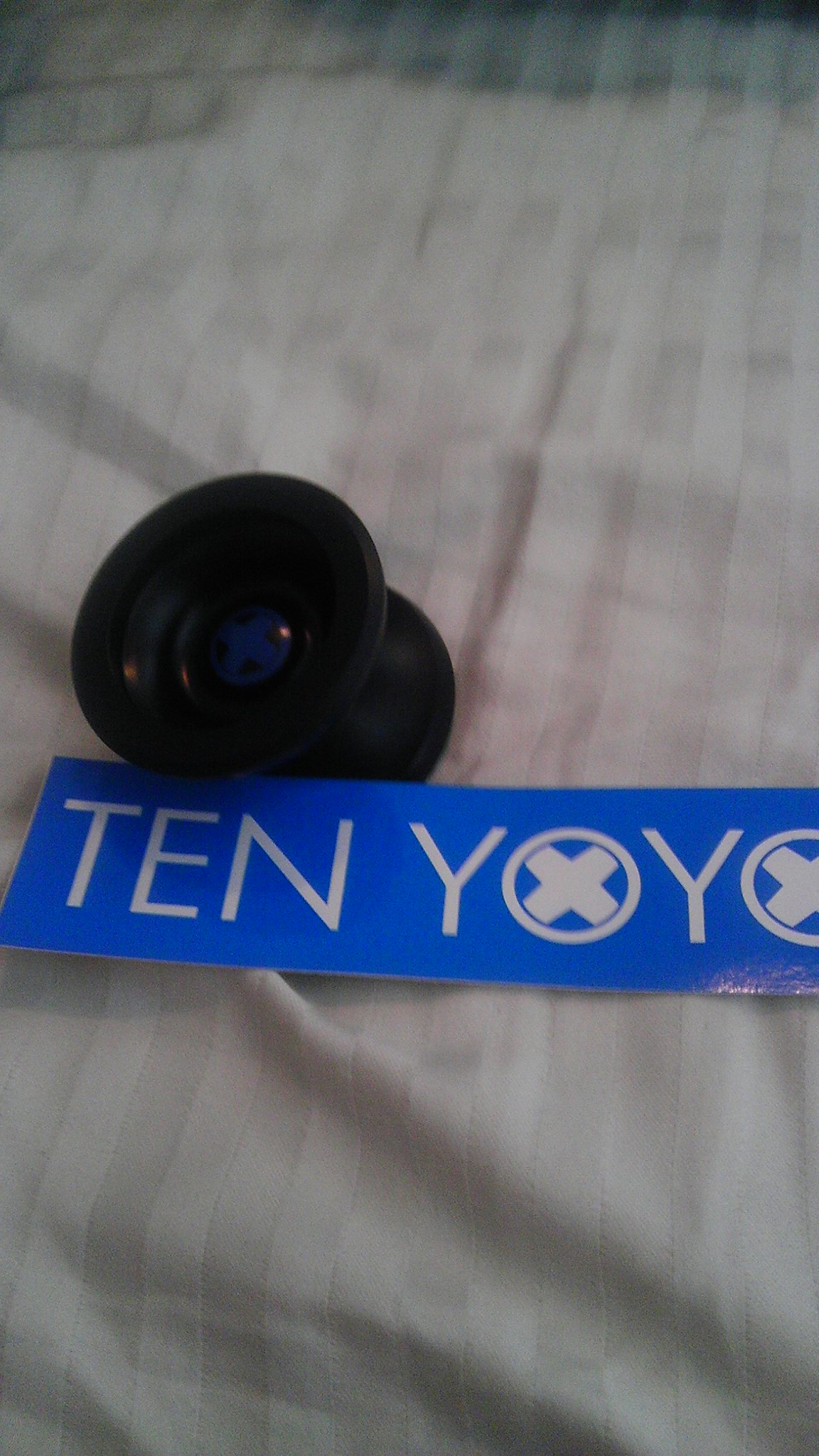The close-up photograph features a black yo-yo with a concave design and a small blue circle at its center, resting on luxurious white striped satin sheets. In front of the yo-yo, there is a thick, rectangular paper tag with a reflective blue surface. The tag is carefully positioned below the yo-yo, displaying the text "Tin Yo-Yo" in bold white font. Notably, the O's in "yo-yo" are creatively stylized with solid white X's at their centers. The overall composition focuses on the sleek design of the yo-yo and the elegantly displayed tag, creating a visually appealing image.